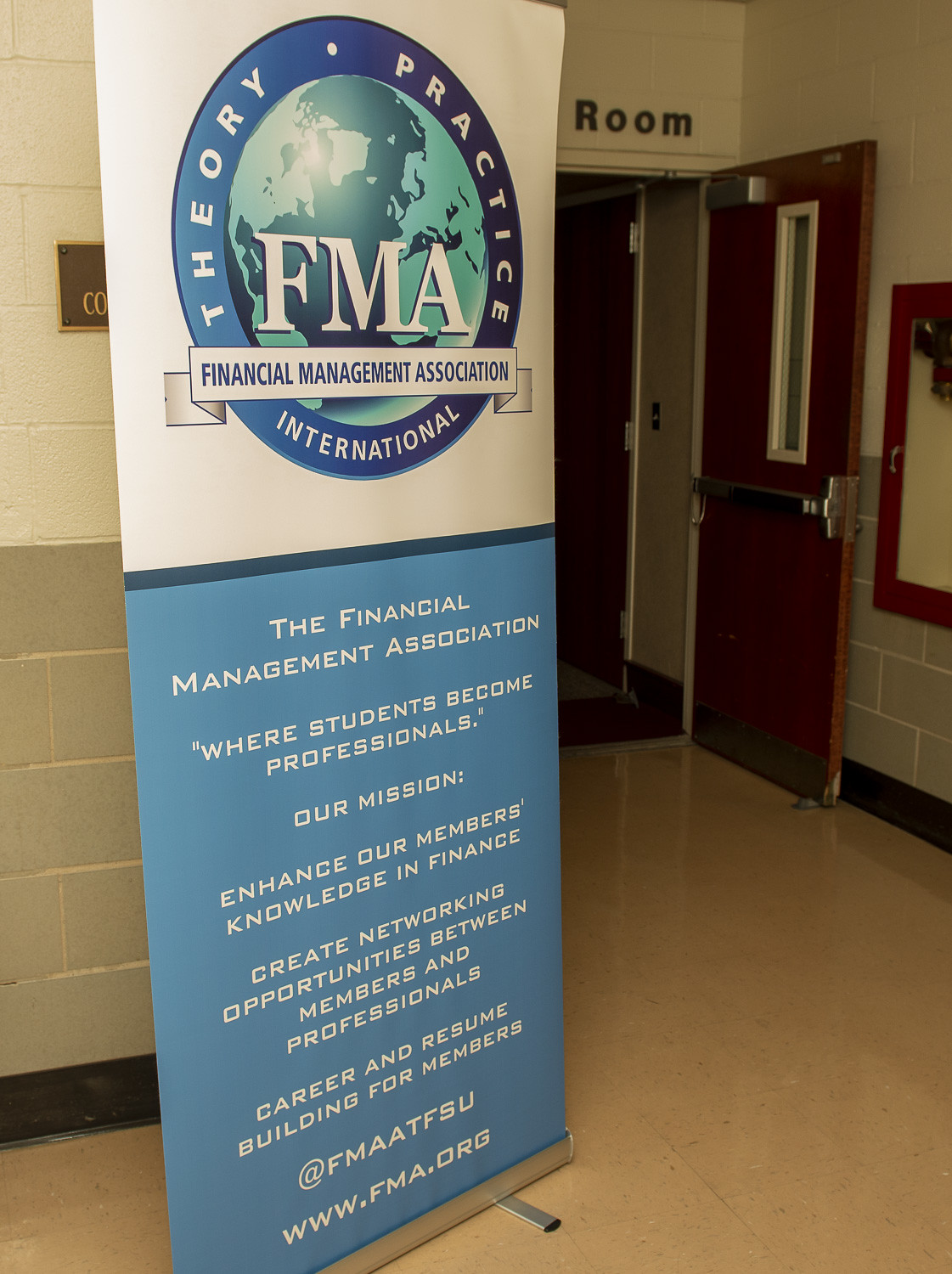The photograph depicts a large vertical banner approximately the size of a door, situated in an office-like space that may be part of a school or educational institution. The room behind the banner has an open door, with the word "room" partially visible above it. The floor is shiny, finished marble, and the wall behind the banner features a light gray, tiled bottom with a white upper section and a black trim at the base.

The banner itself is detailed, showcasing a central circle that contains a globe marked with "FMA." Encircling the globe are the words "Theory Practice International." Beneath this, in larger text, it reads "Financial Management Association," and in smaller text, "The Financial Management Association where students become professionals."

Further down, the banner lists the association's mission: "Our mission is to enhance our members' knowledge in finance, create networking opportunities between members and professionals, and support career and resume building for members." It also includes the website www.fma.org and the specific section at FSU, marked as @FMAATFSU.